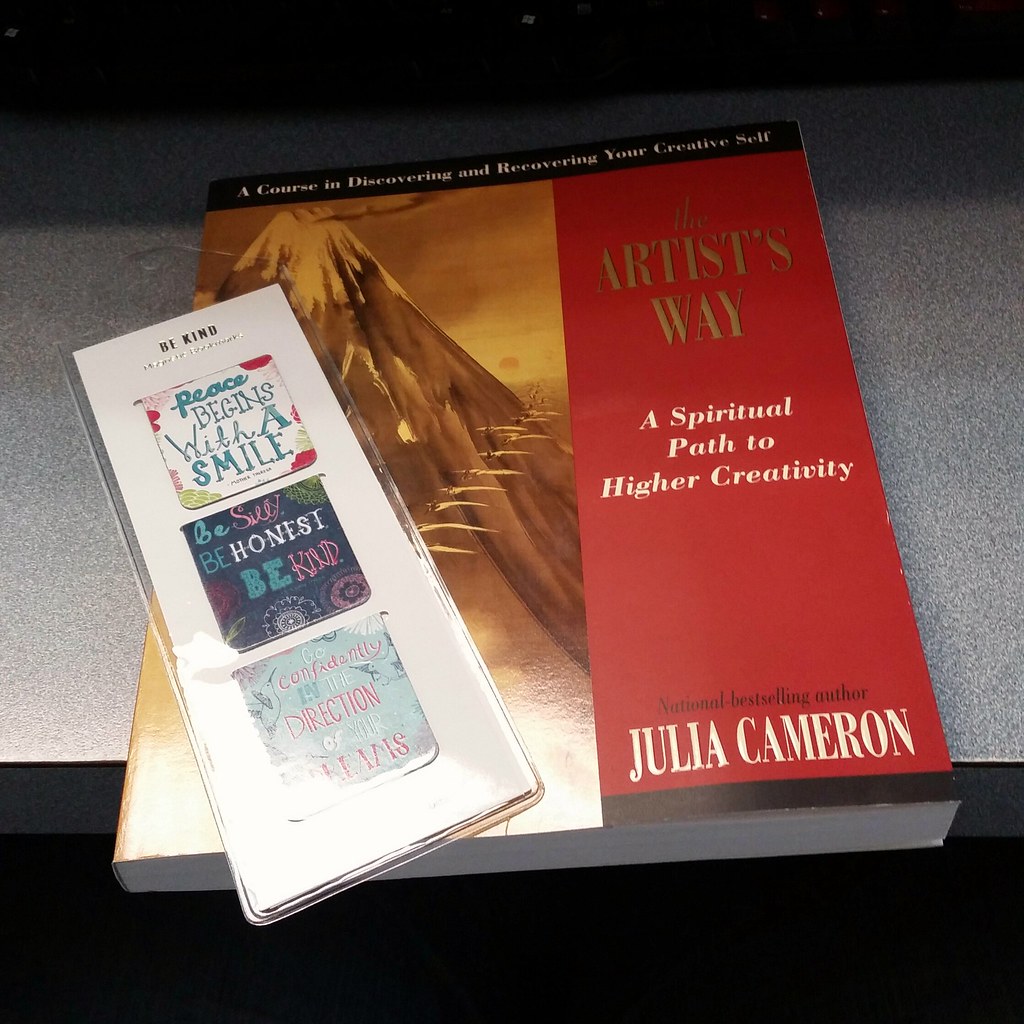The image features the book "The Artist's Way: A Spiritual Path to Higher Creativity" by Julia Cameron, laid on a gray speckled countertop. The book cover displays the title "The Artist's Way" in gold, with the subtitle "A Spiritual Path to Higher Creativity" written in white italics. The top of the cover includes the phrase "A Course in Discovering and Recovering Your Creative Self" in a black banner. Below the author's name, National Bestselling Author Julia Cameron, is prominently noted. The cover also features an orange-themed illustration of a mountain with birds flying towards it.

On the left side of the book, there is a collection of bookmarks placed diagonally in a plastic bag on a white card. The bookmarks display various motivational quotes such as "Peace Begins with a Smile," "Be Silly, Be Honest, Be Kind," and "Go Confidently in the Direction of Your Dreams," though the last word is partially obscured. The speckled gray surface contrasts with the darker black areas both at the top and bottom of the image, adding depth to the scene.